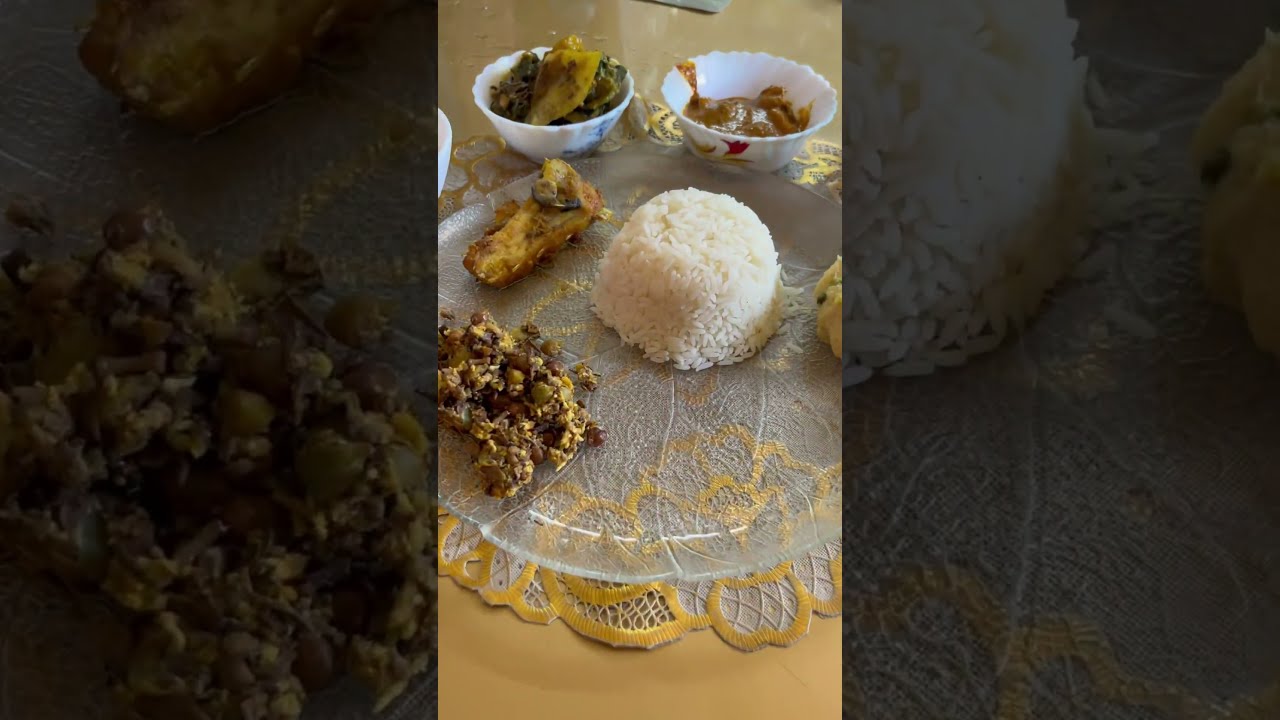In the center of the image, showcased on a gold and cream doily, a large, white mound of rice stands like an upside-down mountain, garnished with a hint of yellow brown on top. Surrounding this focal point are various foods: to the left, brownish dishes, potentially beans and ground items, and a bowl with green elements that resemble broccoli. To the right, a slightly tipped bowl with a brown sauce seeping out, and an unknown brown item adjacent. The scene is set on a tan table. The left and right fragments are close-ups of these details, with the left highlighting the browned food items and the right emphasizing the rice and brown adjacent dish. These side images have a darker hue than the brighter center.